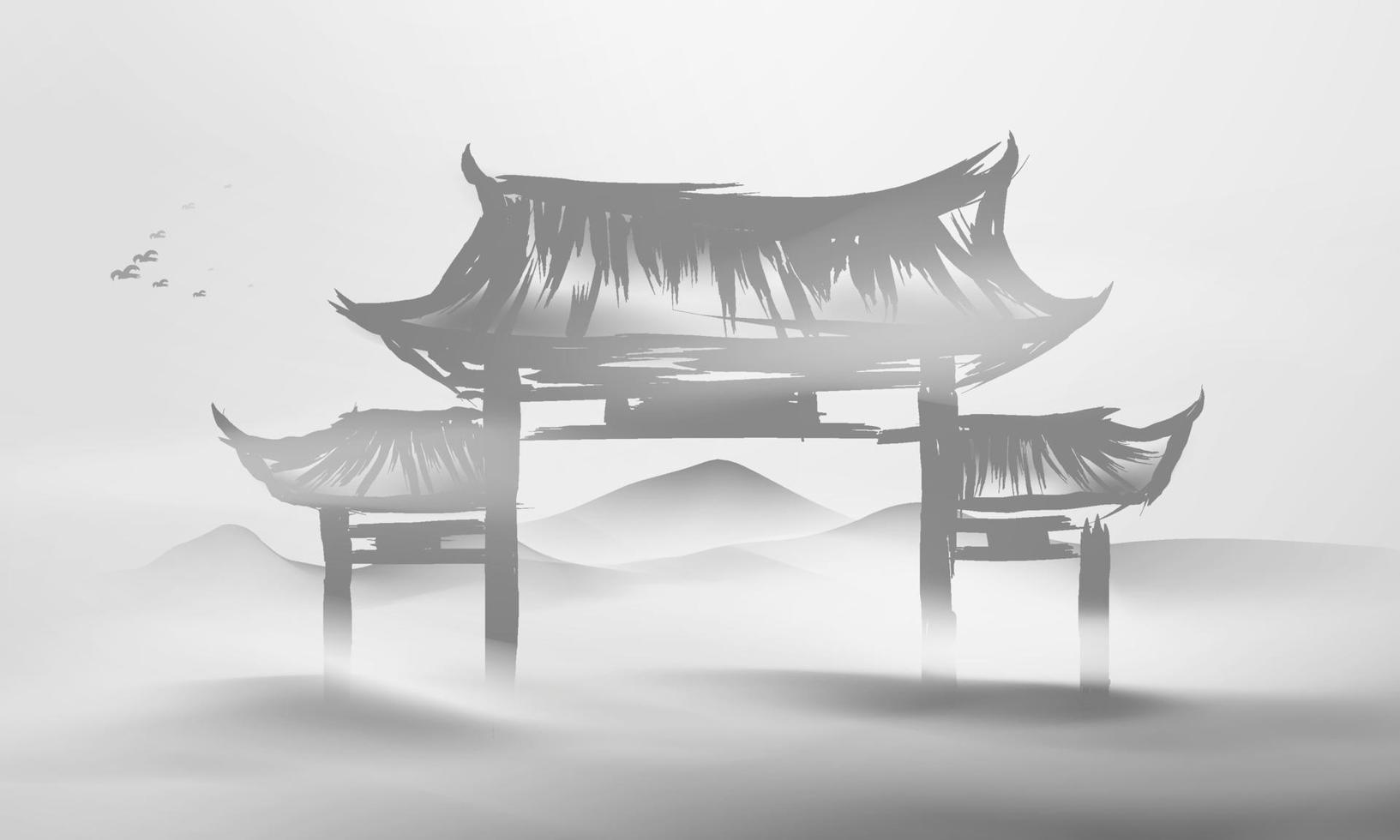This grayscale digital illustration depicts a traditional Chinese pagoda, viewed face-on and centered within the frame. The pagoda features a prominent central section with the tallest roof, supported by four wooden posts. Two smaller sections with matching roofs flank either side, their posts interconnected with the central structure. The roofs and posts are styled to resemble brush strokes or vector art, contributing a textured, artistic feel.

In the background, the silhouette of a mountain range rises to about halfway up the pagoda, with the peaks rendered in darker shades that fade into white at their bases. The sky above is stark white, punctuated by a small flock of gray birds on the left. The foreground features dark shading that gives the impression of mist or fog, enhancing the overall sense of mystery and serenity in the scene. The landscape appears to be covered in a hazy, perhaps snowy, mist, contributing to the tranquil, ethereal ambiance.